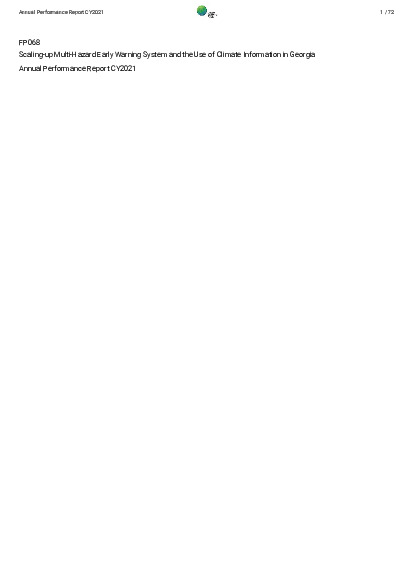In the center of the image, there's a prominent green 3D ball. Adjacent to it, a blurred black icon with potential traces of gray is visible. Located on the far right, "1/72" is faintly decipherable, indicating this is the first page of a 72-page document, though the text is highly pixelated due to extensive resizing.

Towards the upper left corner, the header reads "Annual Performance Report CY2021" in a relatively small font. Below this header, to the left, are the capital letters "F" and "P," and slightly above these letters, the number "068" is displayed. Underneath these elements, a very blurry line of text reads in black sans-serif font, "Scaling Up," followed by "Multihazard Early Warning System and the Use of Climate Information in Georgia." The phrase "Annual Performance" is followed by smaller text indicating "TCY2021."

Overall, the image is of low quality, with significant pixelation making certain details difficult to discern accurately.